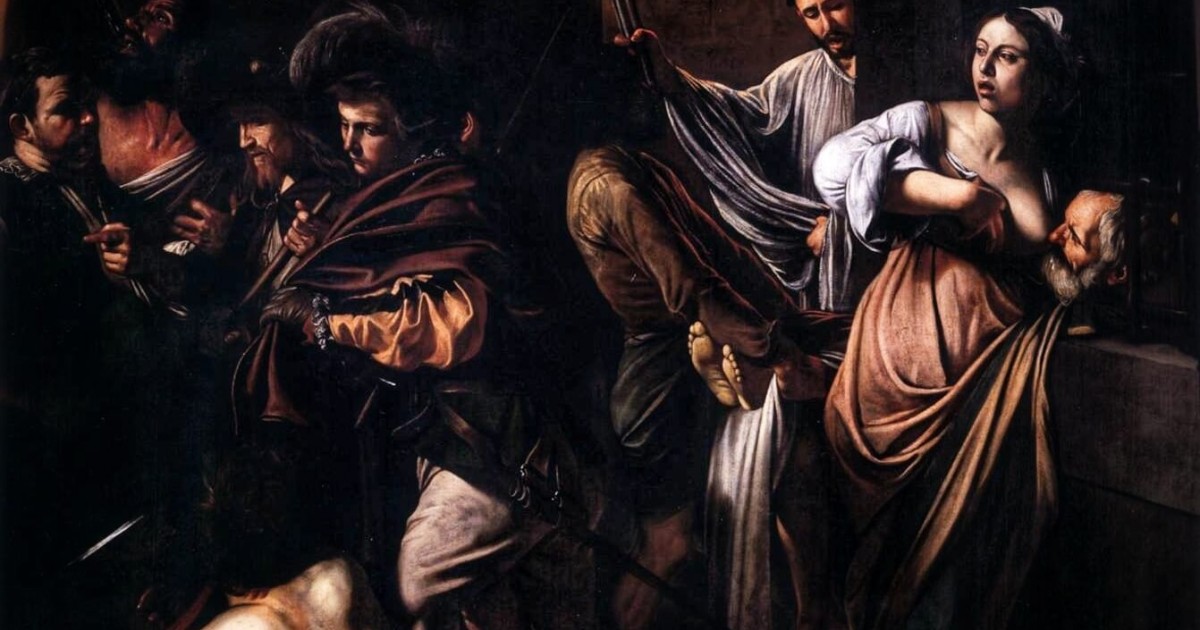The image is a hyper-realistic Renaissance-style painting rendered in dark hues, primarily deep browns, maroons, and beige. On the left side, a group of people dressed in old-timey, Renaissance-era clothing is depicted. In the foreground, a man gazes to the right, while another man stands behind him looking up to the left. To the right of the first man, another individual looks at him while a woman beside this group looks off to the left. The men are attired in loose shirts gathered around the neck and robes draped over them.

In the background on the right side of the image, a table supports a pair of feet, likely indicating a deceased person, with two individuals tending to the feet. Nearby, a woman with one breast exposed stands, accompanied by a man positioned next to her breast. Another male figure in a gown appears to be observing the scene within a darker room, where the feet are being held down. The overall setting is ominous, with light selectively illuminating the figures against the dark backdrop, effectively making them pop out of the encompassing darkness.